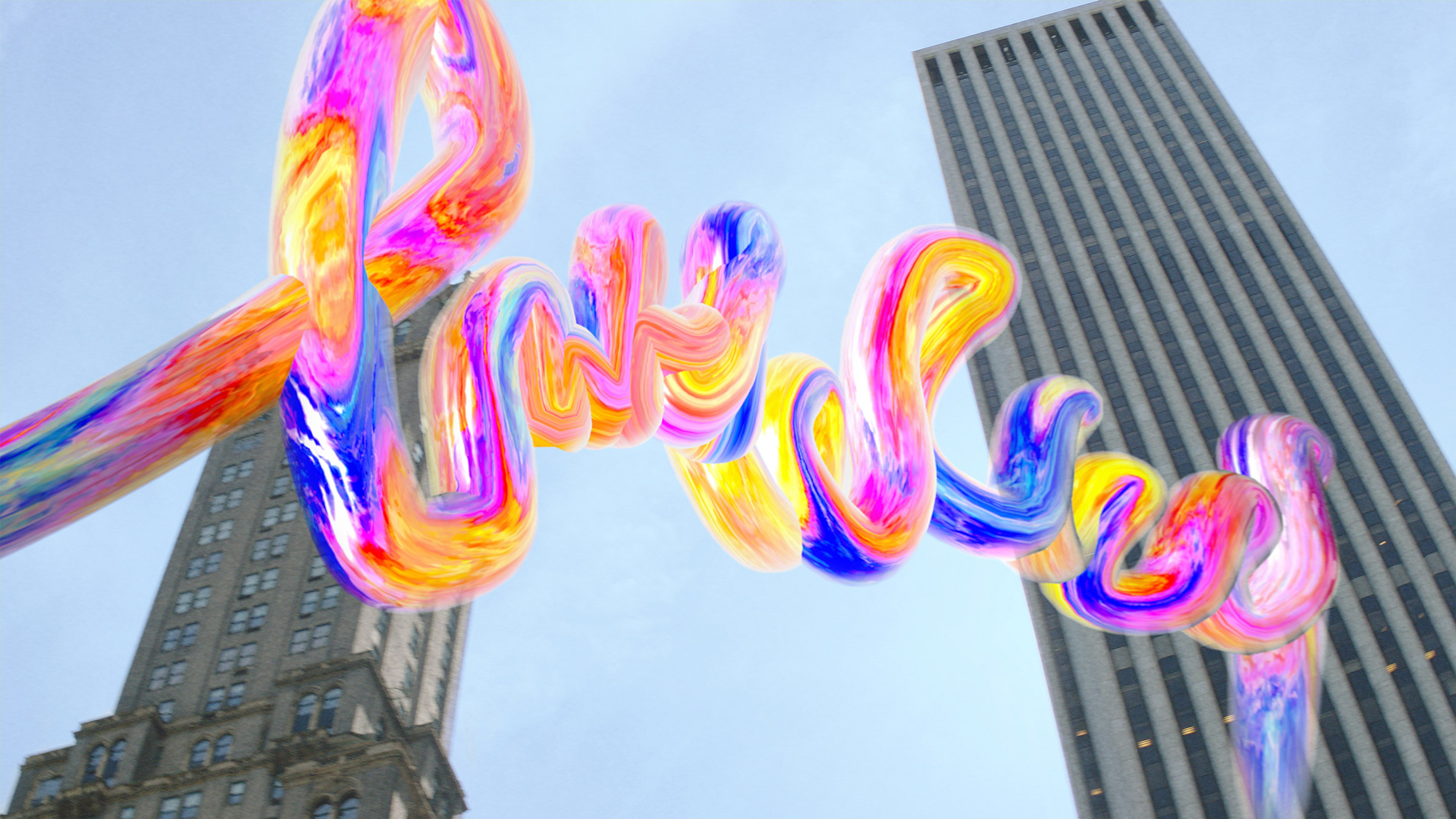This photograph captures an urban scene dominated by two towering skyscrapers set against a predominantly blue sky with minimal cloud cover. The skyscraper on the left-hand side of the image is a light tan color, while the one on the far right is gray and extends all the way to the top of the frame. Central to the image is a striking, multicolored art installation positioned in front of the buildings. This vivid display features an array of bright hues, including blue, pink, yellow, and green, forming a visually captivating pattern reminiscent of a rainbow-colored wave or a series of swirling designs. The display begins on the left side of the image, arches gracefully upward and downward, and continues to undulate across the scene. The photograph, taken from a ground-up perspective, enhances the grandeur of the skyscrapers and the vibrant art installation.